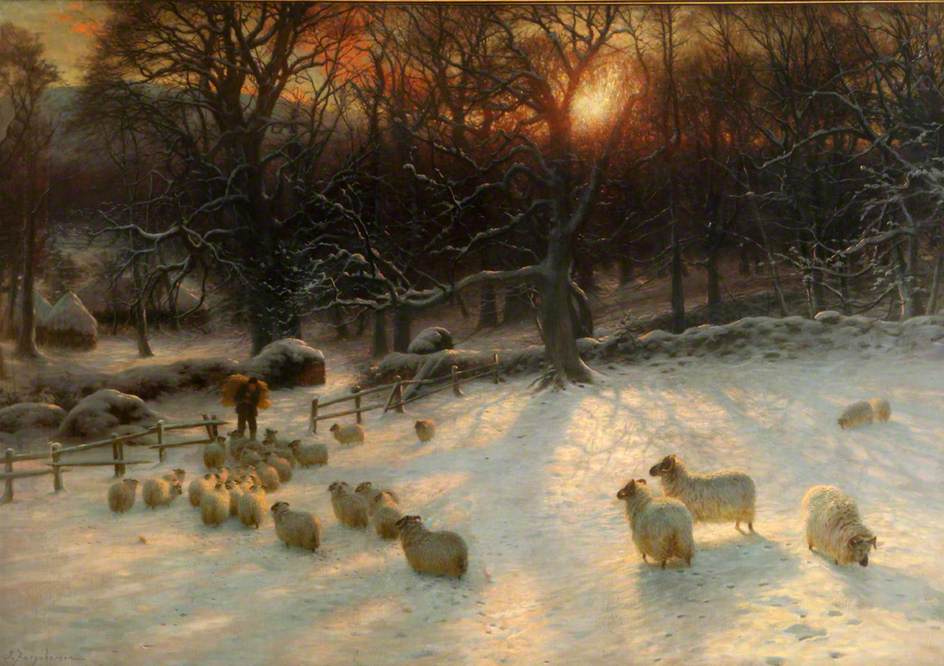In this incredibly detailed painting, we're presented with a serene winter scene. A flock of approximately 25 sheep, characterized by their yellowish and white wool, is gathered within a wooden fence in a snow-covered field. Most of the sheep are clustered around a shepherd who is carrying a bale of hay or possibly wood on his back, and they seem to be following his lead. 

The background is adorned with a dense arrangement of leafless trees, many dusted with snow, adding to the sense of a cold, crisp winter day. To the left, more details unfold with the presence of huts or houses, suggesting a rustic homestead where the shepherd and perhaps the sheep might take shelter. 

The sky above displays a mesmerizing transition from the dark of night to the light of dawn, with an orange sun making its rise, casting a warm glow across the scene. To the left, a mountain quietly stands guard over the tranquil landscape. This remarkable painting captures the harmony between man, animal, and nature in the midst of winter.